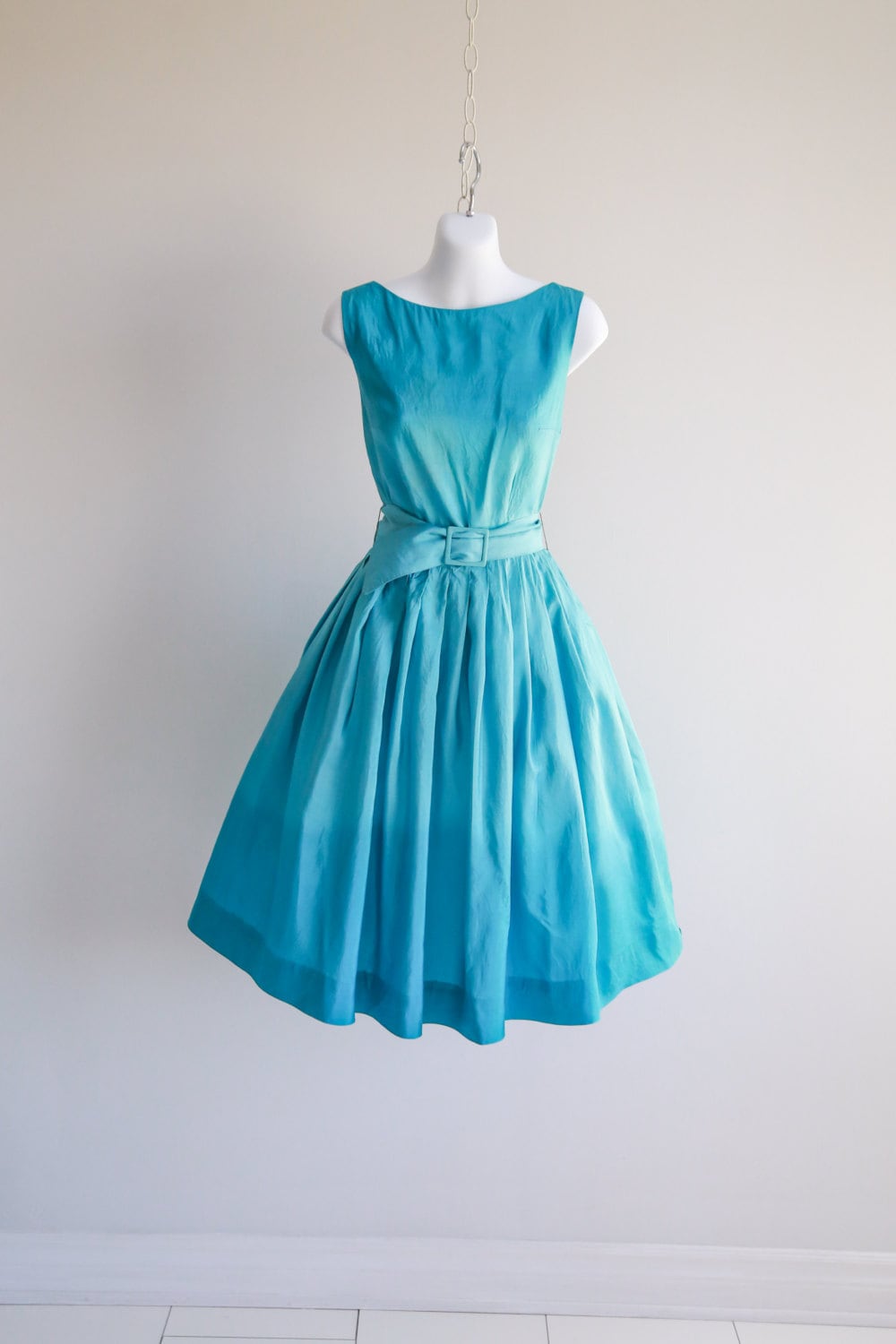This photograph captures an old-fashioned, sleeveless dress in various shades of pastel blue, hanging in a stark white room. The dress, almost translucent yet not see-through, features a boat neck—or crew neckline—with wide straps, presenting a sleek, uncomplicated elegance. The garment is cinched at the waist with a belt of the same material and color, leading into a slightly flared, pleated skirt that ends mid-calf. The delicate fabric showcases a subtle gradient from lighter blue at the belt to darker hues towards the hem, adding a fascinating depth to its design. Displayed on a headless, armless mannequin torso attached to a silver or aluminum chain from the ceiling, the entire scene is rendered against a solid white background with white wooden flooring, epitomizing a minimalist yet vintage aesthetic.